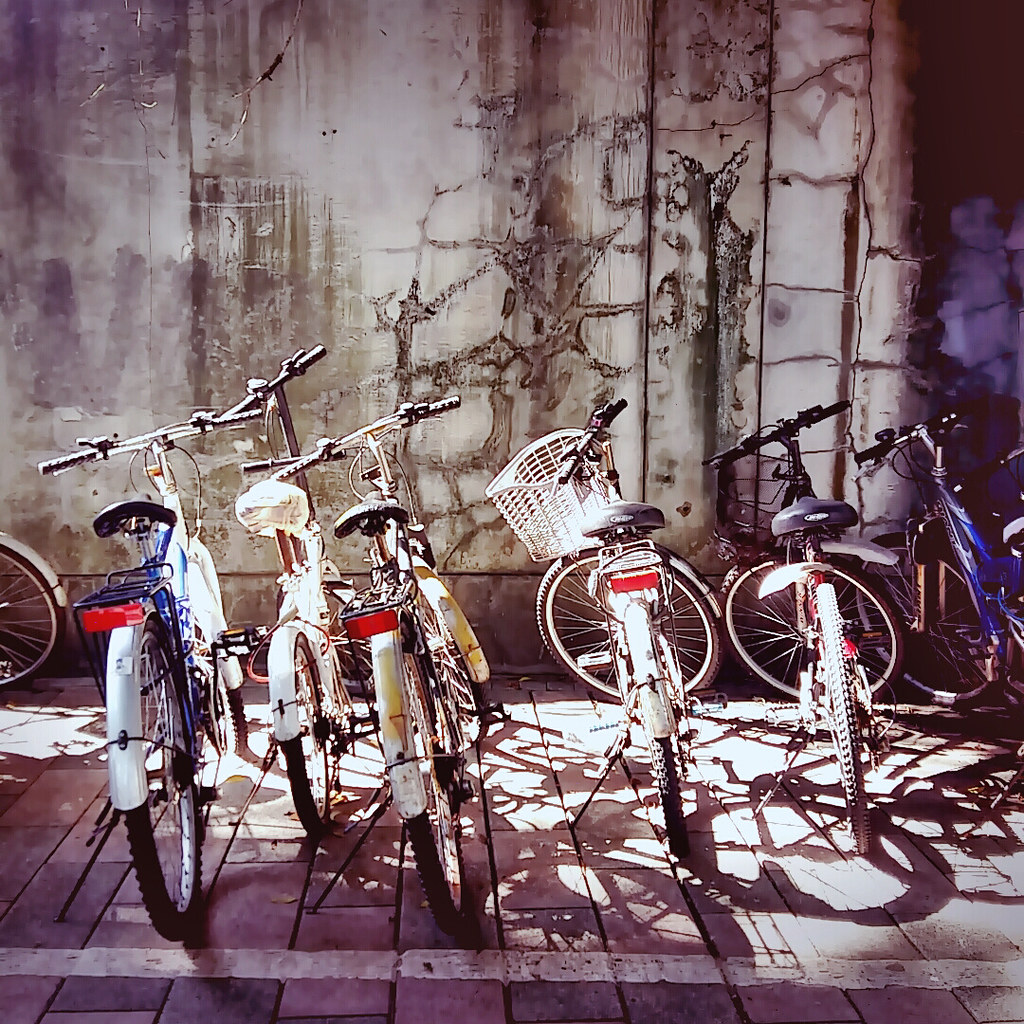The color photograph captures a well-composed image of six bicycles parked side by side on a gray brick sidewalk, with the rear tires facing the viewer. An additional bicycle is partially visible, with only its wheels appearing in the background. Each bike stands on its kickstand, slightly tilted to the left. The bicycles feature predominantly white frames, with some accented in blue and yellow. The tires are black and skinny, framed by sleek silver and white rims.

Notably, all the bicycles have black seats, with red reflectors mounted at the back, suggesting an arrangement for night riding. One bike, positioned slightly right of center, boasts a white wicker basket on its handlebars. The scene is illuminated by sunlight streaming in from the right, casting shadows to the left, thus highlighting the bikes against the aged, weather-beaten concrete wall that serves as the backdrop.

This wall showcases an array of cracks, blackish graffiti shapes, and dark smudges, adding a textured, rustic charm to the setting. Additionally, a conspicuous white line runs across the brick pavement near the back tires of the bicycles, enhancing the overall composition and directing the viewer's gaze through the scene.